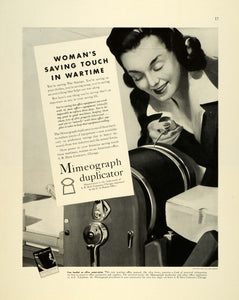This vintage 1950 black-and-white advertisement, possibly from a magazine or newspaper, showcases a woman in a business suit operating a mimeograph duplicator. The background has a cream tint, likely due to aged newsprint. The woman, with coiffed dark black hair, is bent over the round drum of the machine, appearing to add lubricant or ink with an oil can-like tool in her hand. She gazes intently at her task. The ad features a prominent diagonal title, "Woman's Saving Touch in Wartime," accompanied by three paragraphs of text and further elaboration, though these are not legible. The mimeograph duplicator name is prominently displayed at the bottom, along with numerous tiny, unreadable letters. This advertisement captures the essence of the era, highlighting women's contributions in a business setting during wartime.